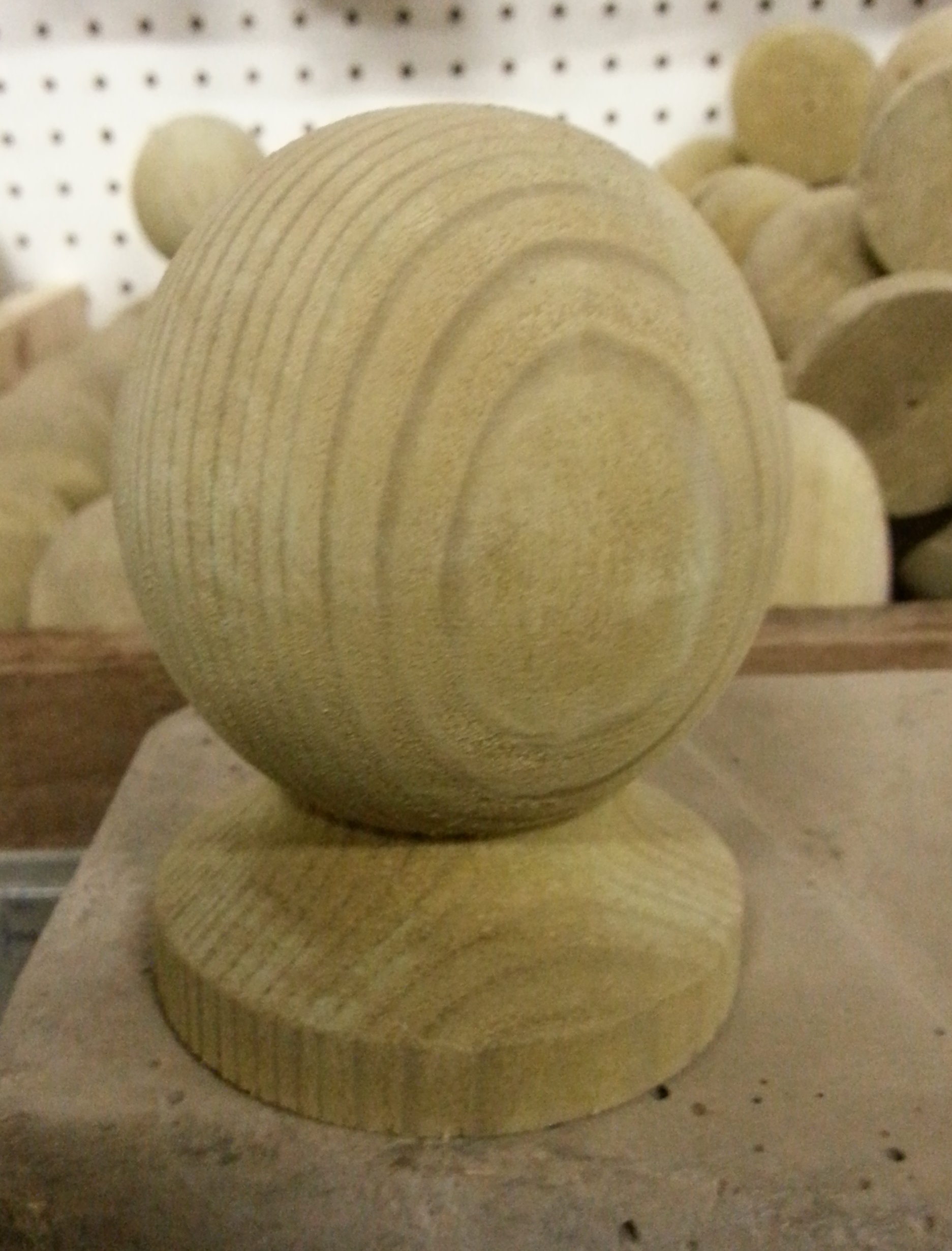This image captures a detailed scene centered around a wooden figure, prominently positioned mid-frame on a brown, possibly concrete-like platform. The wooden figure, which resembles an almost circular wooden sphere with visible grain lines, displays notable craftsmanship with concentric patterns and a light brown hue. The wooden sphere is mounted on a matching wooden base, enhancing its display. Surrounding this figure are multiple similar wooden spheres, scattered and piled chaotically, indicating a collection or storage setting. These additional wooden spheres are situated in what appears to be a wooden box, some piled so high they surpass its edges without falling out. Further back, a white pegboard fills the background, characterized by numerous black-tiny holes designed for peg hooks. This pegboard adds texture and depth to the scene, contrasting with the wooden elements present.